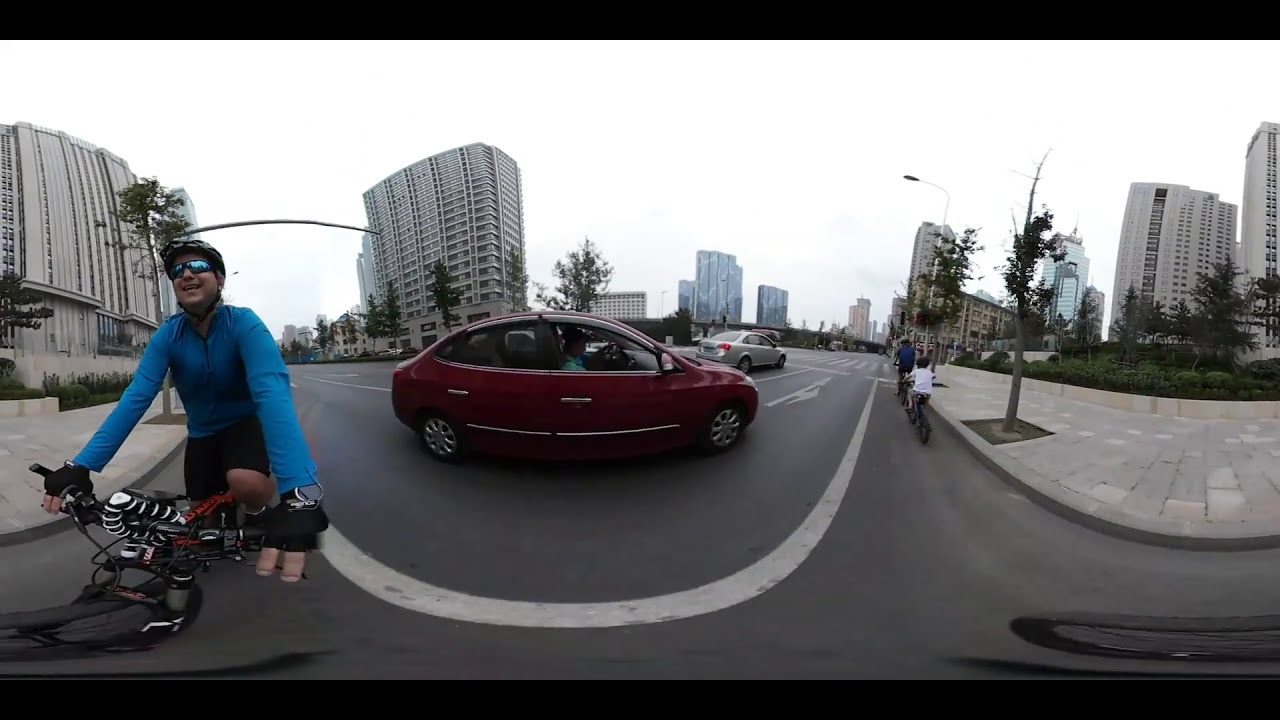In this dynamic fisheye lens photograph taken in an urban setting, a smiling man in a long-sleeve turquoise blue zip-up tracksuit and black biker shorts is the focal point as he rides his bicycle towards the camera. He dons reflective turquoise-tinted sunglasses and a black helmet, and both his hands are firmly placed on the handlebars. The warped curvature of the gray concrete road with its white markings adds a distinctive visual flair, curving like a smiley face. A red maroon sedan with black wheels is captured making a turn to the right, adding a sense of movement to the image, while a gray car is visible further behind. In the background, a mix of tall buildings and skyscrapers, along with lush green trees, frame the scene, providing a bustling city ambiance. Off to the right, an adult and a child are seen cycling away, while the sky above them appears glary white. The photo is bordered by relatively thick black margins at the top and bottom, which enhance the framing of this vivid urban street scene.